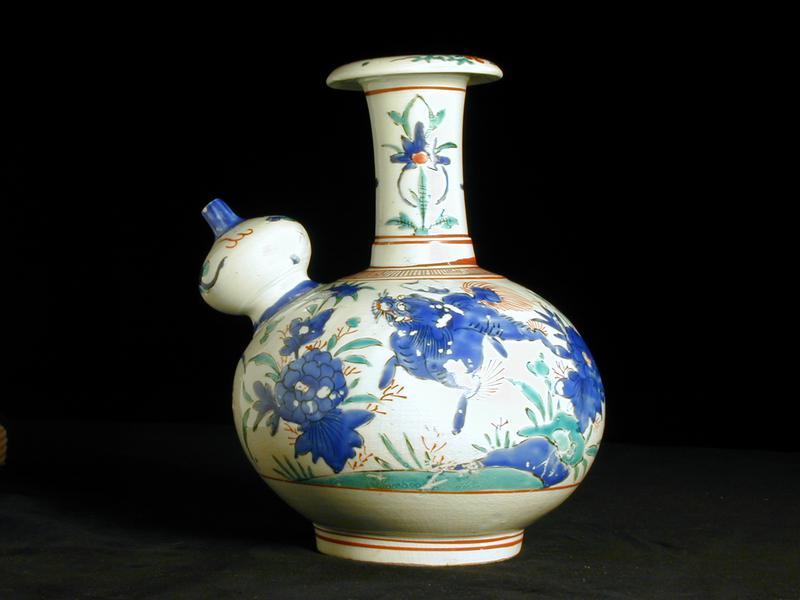The image showcases a white ceramic teapot or pitcher with a meticulous and ornate design set against a black background. The body of the teapot, situated in the middle of the image, features a bulbous, oval shape adorned with intricate blue floral patterns, light blue leaves, and small brown twigs. Among the decorations is a striking blue dragon, seemingly swimming towards the upper left of the vessel. The base of the teapot displays red stripes, creating a contrast against the predominantly white surface. Rising from the center is a cylindrical stem that flares out at the top and is capped off with a flat, rounded lid. This stem area is also decorated with blue flowers and green leaves. Extending from the upper left of the teapot is a short, spouted extension with a rounded body that tapers to a white tip accented in blue. The entire scene is set against a grayish-black surface, providing a dramatic backdrop that highlights the delicate and detailed craftsmanship of the teapot.